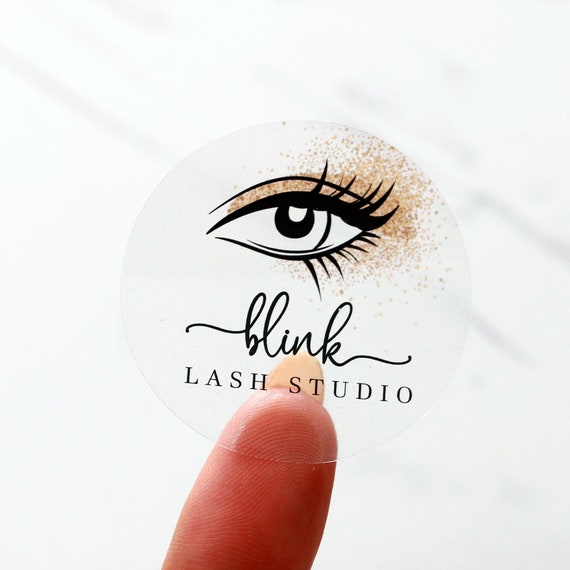The image showcases a marketing flyer with an all-white, slightly rough background. At the bottom of the image, a person's finger—marked by visible fingerprints and a long nail—presses against a transparent sticker. This sticker features a detailed illustration of an eye, complete with black eyelashes, black eyebrows, and a black cornea. Surrounding the eye are yellow spots, possibly representing makeup. Below the eye, the text "BLINK LASH STUDIO" is written in black, with "BLINK" in cursive and "LASH STUDIO" in all capital letters. The background also includes some subtle gray lines, adding texture to the overall image.